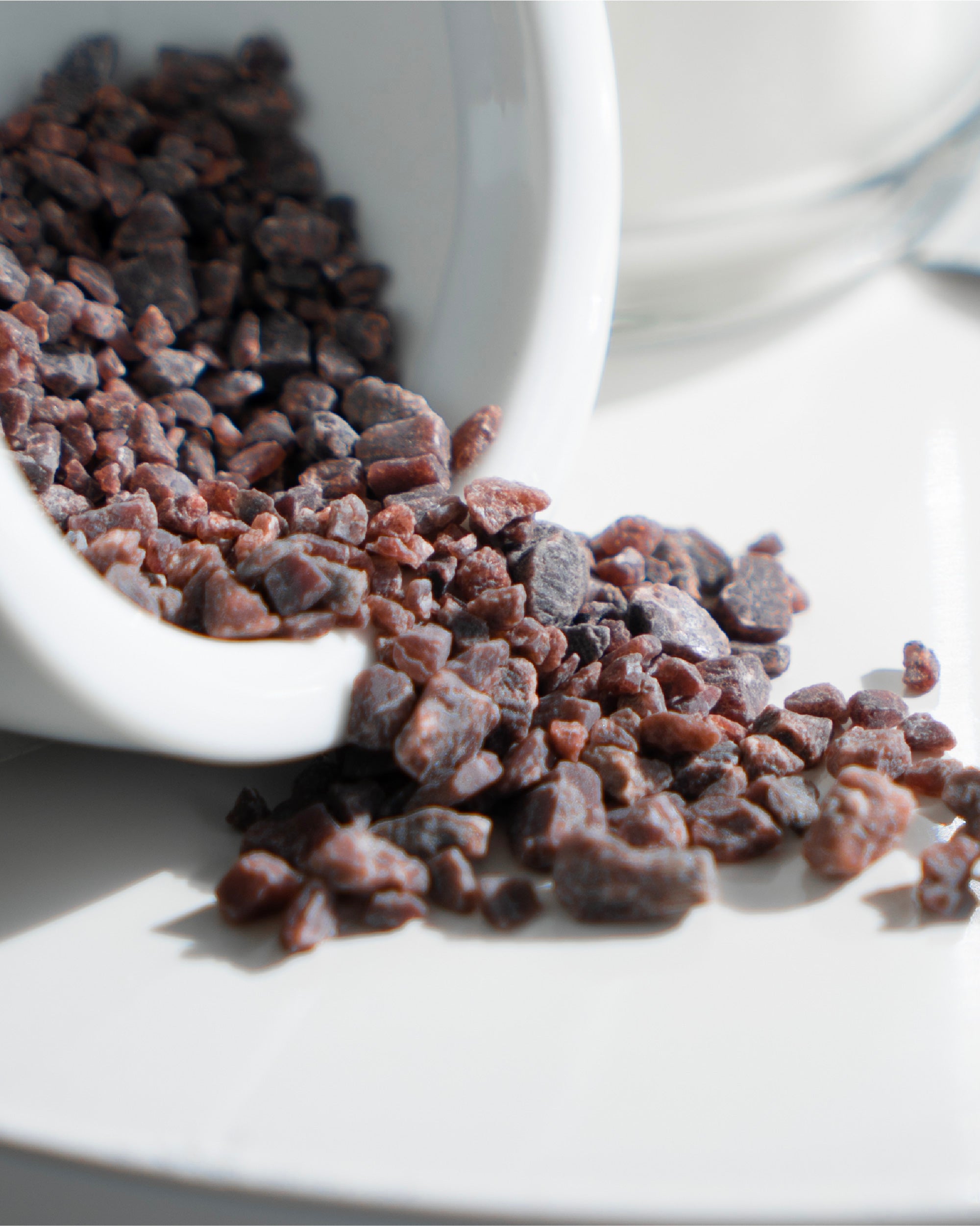In this image, a white bowl is tipped over on a white tabletop, spilling its contents. The bowl appears about halfway full with small, dark red to black rock-like objects, resembling either dog food, small pebbles, or perhaps agates. These objects vary in size but are generally small, comparable to acorns or gravel. The predominant colors in the image are the stark white of the bowl and table contrasted by the burgundy hue of the spilled contents. Shadows cast by the bowl and the objects add depth to the scene. In the background, there is a faintly visible blurry object with a small blue line descending from the upper right, suggesting another plate or bowl is present but not the focus of the image. The overall effect is one of neat simplicity, highlighting the contrast between the white surface and the dark, scattered contents.